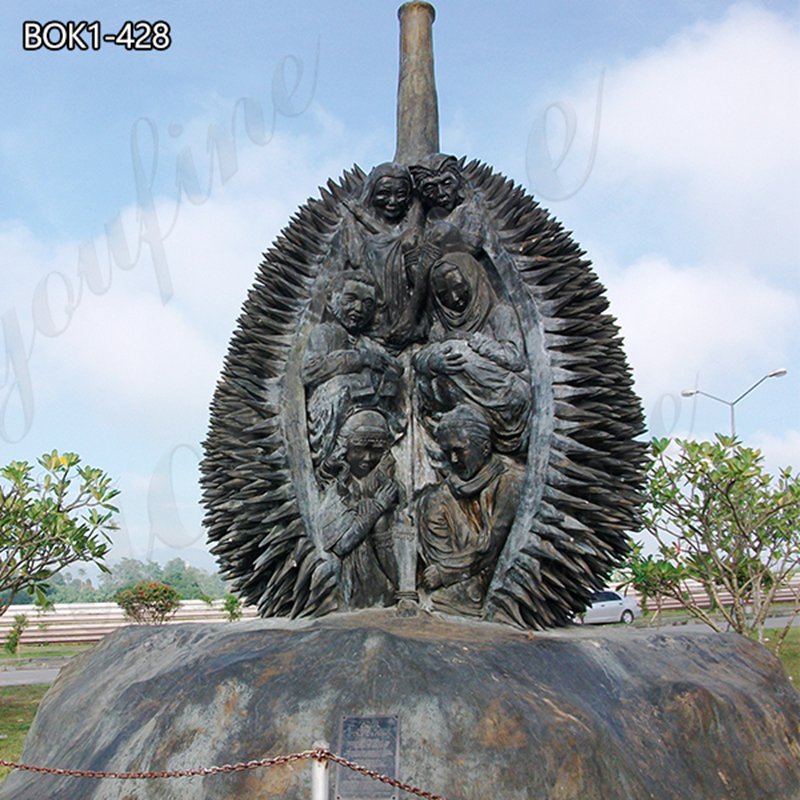This outdoor photograph, likely a professional piece, captures a striking stone sculpture prominently positioned at the center of the image. The sculpture, resembling a large, spiked fruit akin to a durian or pine cone, stands atop a larger stone pedestal. Intricately chiseled, this gray stone formation features lifelike carvings of approximately six to eight individuals, some seemingly indigenous. The figures include a woman with a baby and another person draped in a veil, each figure detailed with various expressions and postures.

Surrounding the sculpture, a metal chain link fence prevents visitors from approaching too closely, while a small, weathered placard attached to the stone base remains unreadable from the distance. The background features a clear, daytime sky with scattered white clouds, lush green trees, a roadway, and partial views of cars and streetlights, suggesting a park setting during spring or summer. The image is watermarked with "joufine" and marked with "BOK1-428" in the upper right-hand corner.